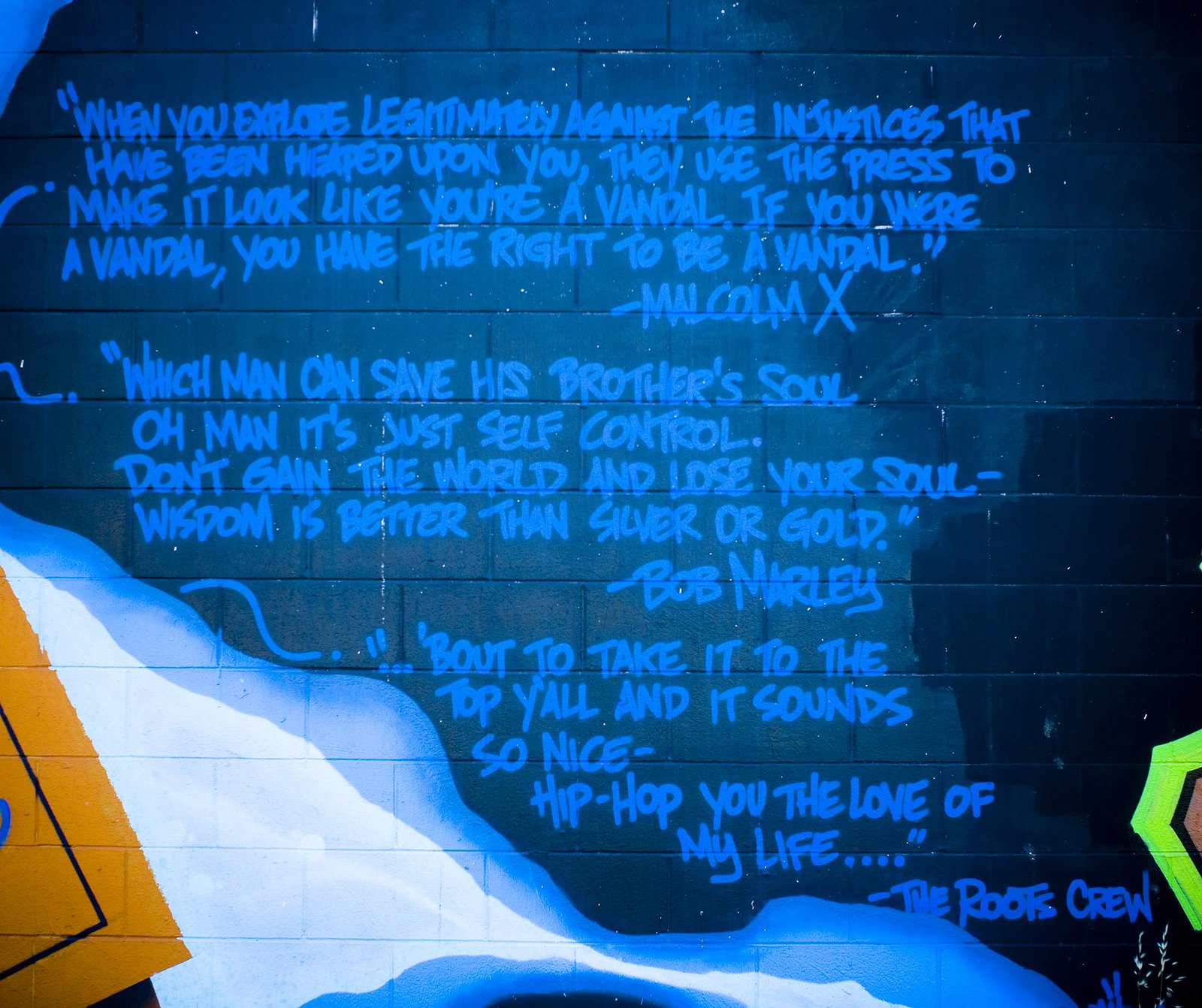This image captures a vivid piece of street art on a cinder block wall painted in a dark navy blue, splashed with white specks to resemble stars. The artwork features handwritten, brush-painted quotes in blue text from notable figures and groups, conveying messages about justice, wisdom, and music. The quotes include:

- Malcolm X: "When you explore legitimately against the injustices that have been heaped upon you, they use the press to make it look like you're a vandal. If you were a vandal, you have the right to be a vandal."
- Bob Marley: "Which man can save his brother's soul? Oh man, it's just self-control. Don't gain the world and lose your soul. Wisdom is better than silver or gold."
- The Roots: "About to take it to the top, y'all, and it sounds so nice. Hip-hop, you the love of my life."

The wall also features artistic streaks of blue and white paint, primarily at the bottom part of the image. In the bottom left corner, there is a distinct orange box, adding a vibrant contrast to the overall blue theme. The artwork's raw, painted texture adds to its street art authenticity, blending powerful words with visual appeal.